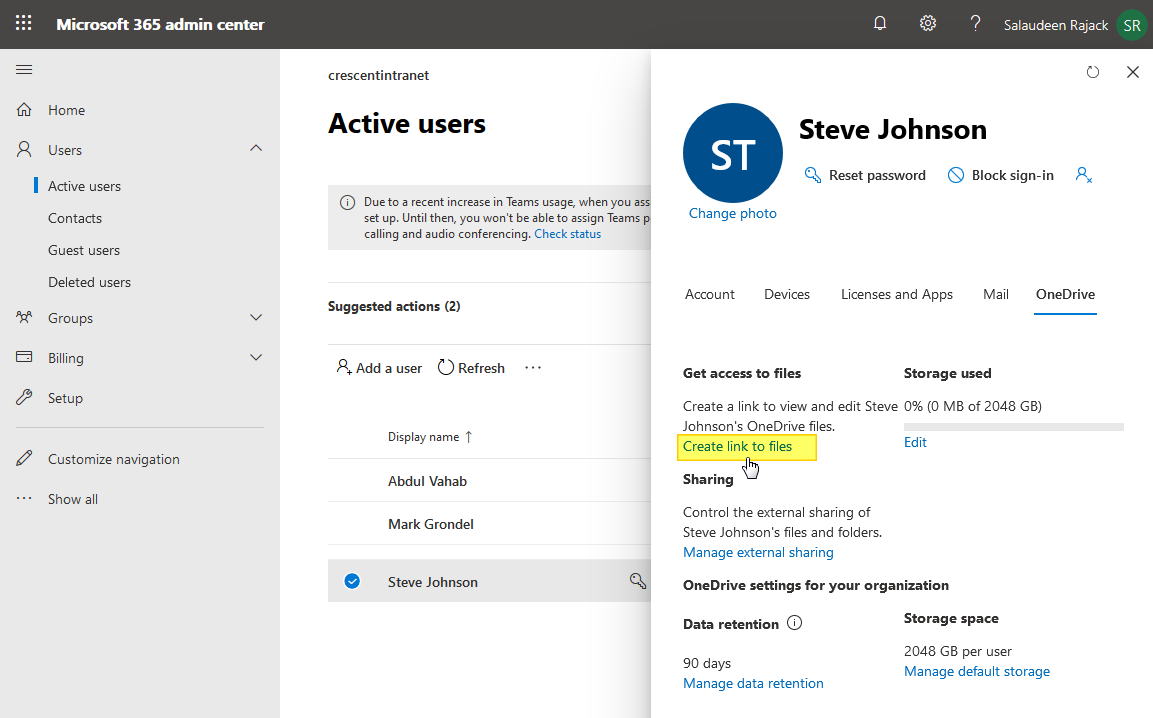In the image, the user is navigating the Microsoft 365 Admin Center. The interface is divided into several distinct sections:

1. **Left Navigation Pane:** This pane includes various administrative options such as Home, Users, Groups, Billing, Setup, Customize Navigation, and Show All. The user has expanded the 'Users' section, revealing sub-options like Active Users, Contacts, Guest Users, and Deleted Users. They are currently focused on 'Active Users'.

2. **Main Content Area:** The main section of the page displays the 'Active Users' list. At the top, there is a header with the title "Crescent Intranet". Beneath this, there is a message addressing the recent increase in Teams usage, followed by a note regarding calling and audio conferencing, which is partially obscured.

3. **User Details Pane:** When the user clicked on Steve Johnson's name from the Active Users list, a detail pane for Steve Johnson opened on the right side of the screen. This pane provides several options for managing Steve Johnson’s account, including adding a photo, resetting the password, blocking sign-in, and accessing files. It also shows that no storage has been used by this account, indicated by 'storage used'.

The interface appears to be used for managing different aspects of user accounts within the organization’s Microsoft 365 environment.